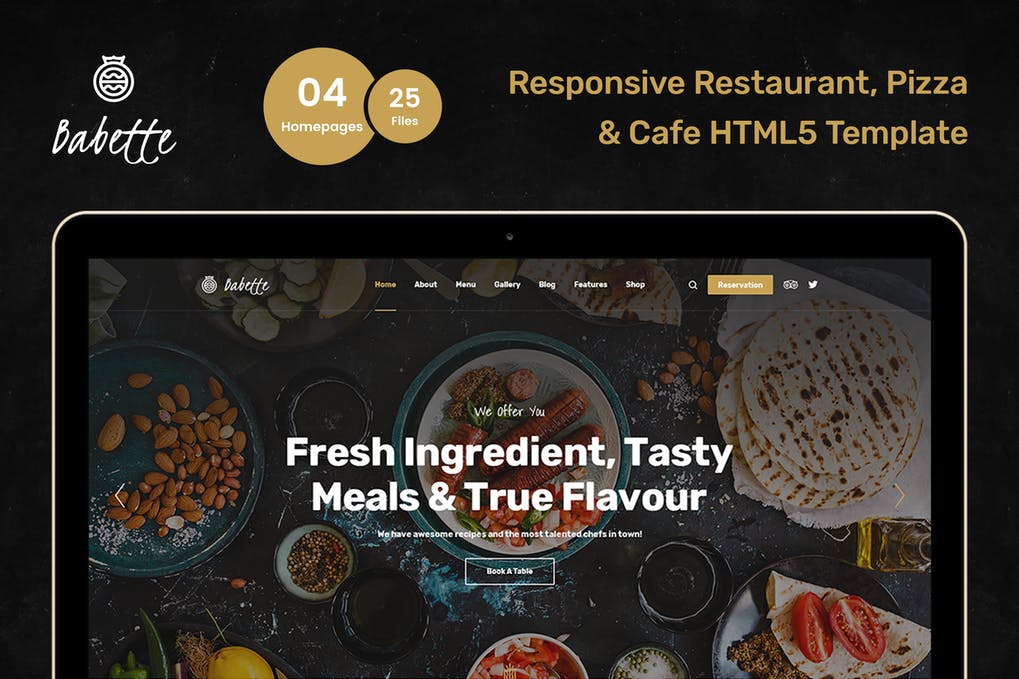The image showcases a sleek, modern restaurant website template, dominated by a rich black background. At the center, a computer screen displays the template. Above the screen, to the left, the word "Babbit" is elegantly scripted in a cursive font alongside a logo. To the right, a prominent yellow circle displays "0" indicating home pages, followed by a smaller circle indicating "25 files." Adjacent to these circles, yellow text reads, "Responsive Restaurant, Pizza and Cafe HTML5 Template."

Below the descriptive text, the template suggests its association with "Babbit," presumably the restaurant’s name. The navigation bar at the top includes icons and links labeled Home, About, Menu, Gallery, Blog, Features, and Shop. It also features a search icon and a prominent yellow "Reservation" button, accompanied by a few subtle logos.

The overall image is set against a culinary-themed background viewed from above, featuring an assortment of foods such as tortillas, nuts, tomatoes, various seasonings, and bowls of ingredients laid out on a table. Stretching across the top of this background, white text declares, "We offer you fresh ingredients, tasty meals, and true flavor. We have awesome recipes and the most talented chefs in town." Beneath this text, a transparent white button invites users to "Book a Table."